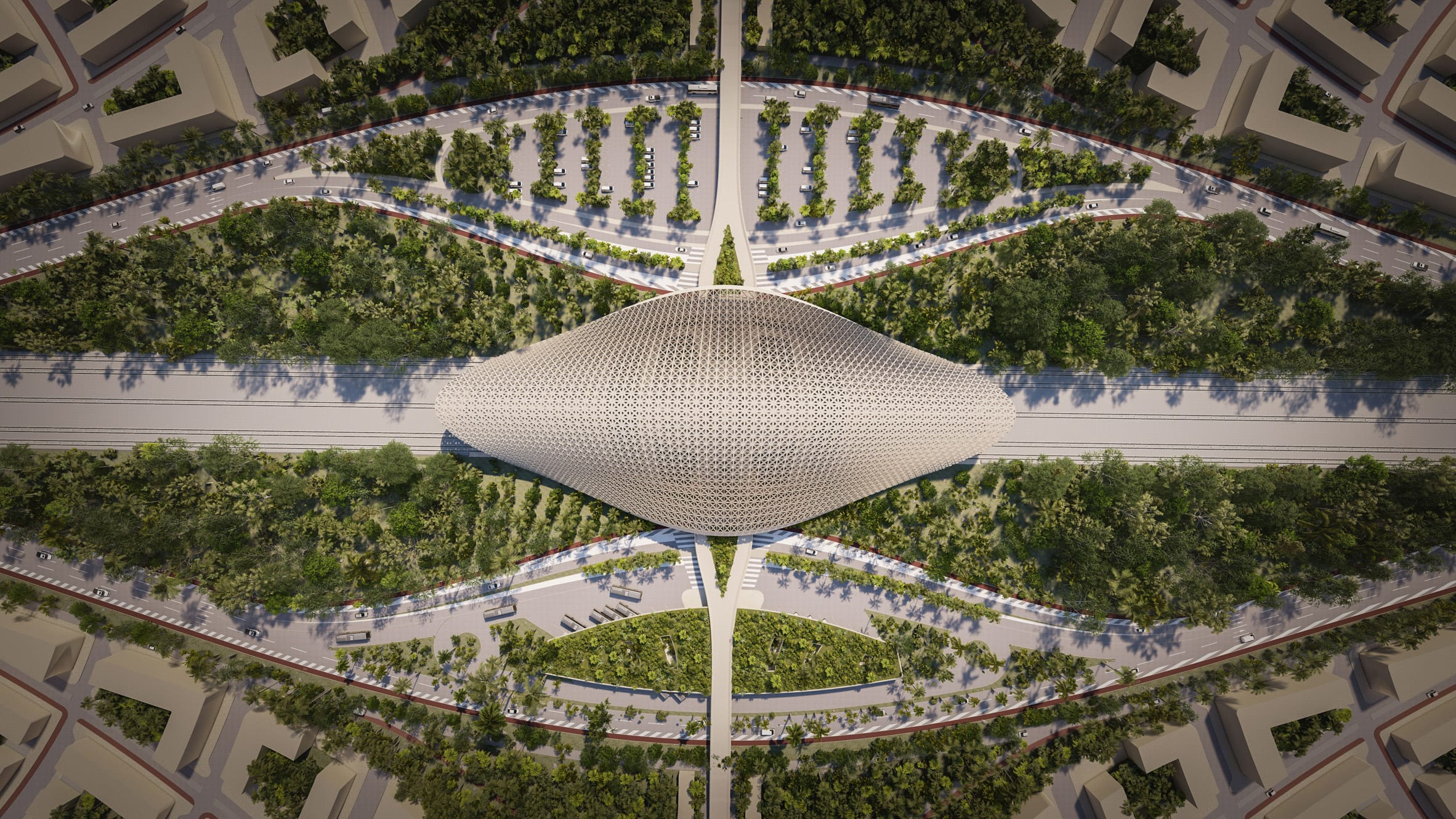This image appears to be a detailed bird's-eye view of a planned urban area, possibly a digital rendering intended for a planning commission. The focal point of the image is a large, oblong-shaped domed structure or cupola situated in the center. This dome is surrounded by a mesh-like covering, creating a distinctive shape that is thick in the middle and tapers off towards the sides. A significant roadway or pathway runs horizontally across the middle of the image, intersecting the domed structure and leading off the edges of the frame.

The image features multiple L-shaped and U-shaped structures scattered around, particularly noticeable in the upper left and right-hand corners, as well as the bottom. These structures are interspersed with a wealth of green trees, creating a lush, green environment. There are clearings with trees positioned between the lines forming the L-shapes, emphasizing the integration of nature within the urban design.

Several pathways and roadways branch off from the central roadway. One such pathway starts at the top middle and extends downward, possibly a sidewalk or smaller road. Another curved path begins in the top left, winding its way up and to the right before curving back down. Smaller branches diverge from these paths, further contributing to the network of roads and pathways.

The image captures the essence of a highly planned, green urban area, with trees and vegetation prominently featured throughout the spaces between structures and roads, adding a natural aspect to the urban landscape. Additionally, some areas seem to contain parking spaces, blending functionality with aesthetic considerations.